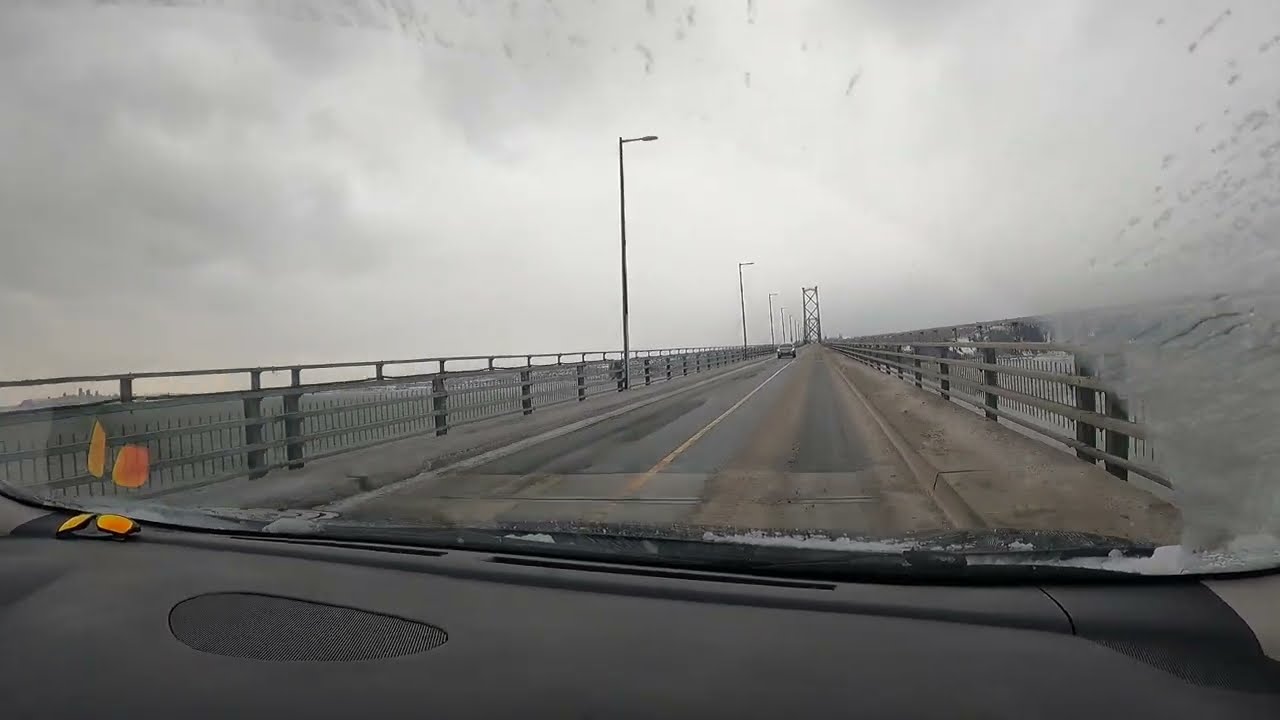This image captures a stormy, overcast scene from the perspective of a driver inside a vehicle traveling over a bridge. The photograph is taken through a windshield that has a murky buildup of ice, snow, or rain, with clean streaks clearly demarcated by the path of the windshield wipers. The road ahead is dark with brown streaks, and the dashboard inside the car is black. There are solid yellow lines dividing the two lanes on this side of the bridge, which suggests traffic flows in both directions with two additional lanes to the left, separated by a metal railing. The right side features a metal sidewalk railing, and you can discern lampposts lining the bridge. Water is visible on either side of the structure, and buildings can be seen distantly to the left. A prominent metal support structure or tower rises at the far end of the bridge, adding to the scene's industrial feel. The overall atmosphere is dominated by heavy gray skies, reinforcing the impression of inclement weather.